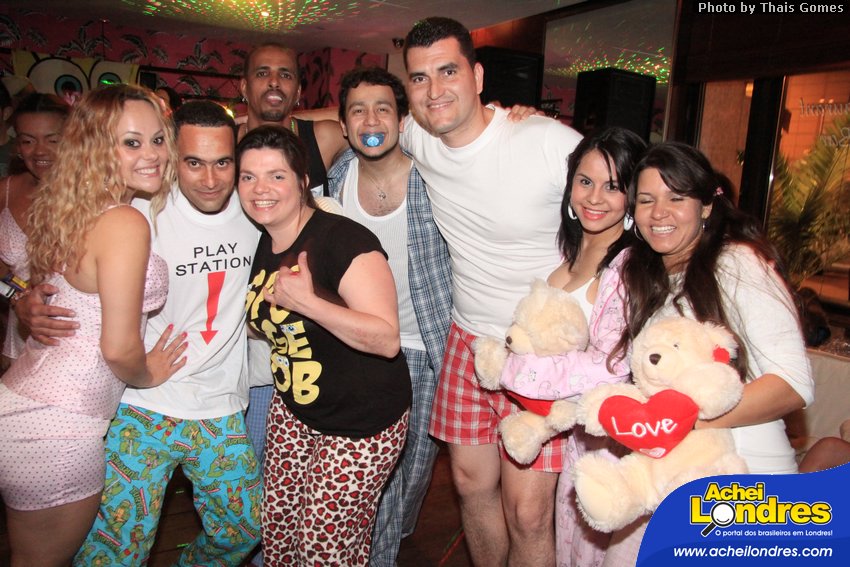The photograph captures a lively gathering, likely a pajama-themed party, showcasing a group of nine men and women posing for the camera. On the far right, two women with long brown hair are holding light yellow teddy bears, each clutching a red heart-shaped cushion with the word "love" written in white. One of these women is dressed in a pink pajama robe and has white earrings, while the other appears to be wearing a white gown with her eyes closed. In the center stands a tall man smiling broadly in a white T-shirt and red checkered shorts. Directly beside him is a shorter man, distinctive with a blue pacifier in his mouth, donned in a white singlet and blue plaid pajamas, suggestive of a fun and light-hearted vibe. In the foreground stands a woman wearing red heart-printed pajama bottoms and a black SpongeBob T-shirt, her brown hair pulled back and a smile illuminating her fair-skinned face. She’s affectionately hugging a darker-skinned man in a white PlayStation T-shirt and blue pajamas. Next to him, on the far left, a blonde curly-headed woman is dressed in a pink silk sleeveless top and shorts, maintaining a playful pose with her hand touching the man’s waist. The background glows with lights, setting a festive atmosphere, and the scene is marked by the text "Ache Londres, WWW.ACHEILONDRES.COM" at the bottom right of the image.